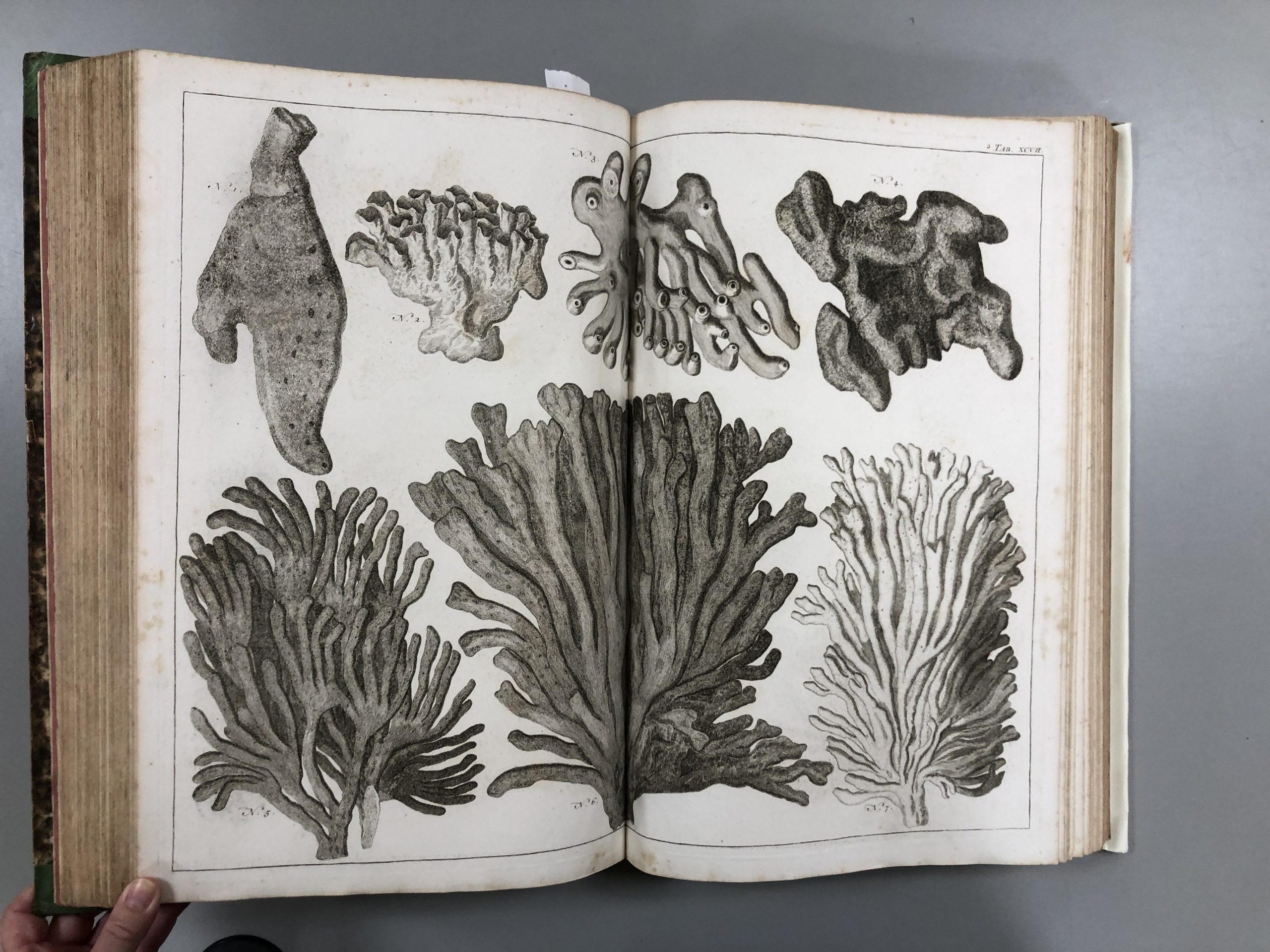In this photograph, an aged book lies open on a glossy, light gray surface, appearing quite old with its browned, worn edges. The creamy white pages are slightly yellowed, indicative of antiquity. The spine and back cover are brownish-tan with dark green and mottled black patterns visible on the left side, while a portion of the right side's cover peeks out, showing a white edge. The book is held open by a thumb and index finger, visible in the bottom left corner of the image.

Spanning across both pages is a continuous, detailed black-and-white illustration, consisting of seven distinct sea plants. The top row features four smaller, spongy-looking plants, while the bottom row showcases three larger, bushy plants with rounded leaves or stems. Among these, the third plant on the bottom row is notably lighter in color, almost white. A small black border demarcates the edge of the illustrations on both pages. Additionally, small black writing is seen in the top right corner of the page.